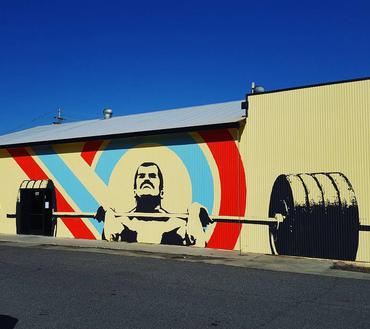The image, taken outdoors during the day under a clear medium blue sky, features a prominent wall mural on the side of a wide, corrugated steel building. The corrugation provides a textured backdrop of vertical lines that bend in and out, enhancing the mural's visibility. In the foreground, there is a paved asphalt road. The mural is the focal point and depicts a silhouette of a man with dark hair and a mustache, lifting a barbell loaded with four large weights on each side. The lifter's pose suggests he is in the midst of a challenging push press, with the bar positioned just under his chin. The background of the mural is a light yellow, matched to the building's color, and features a distinctive logo-like design. Surrounding the lifter, a red stripe curves from the left, looping down and around to form an incomplete circle. Inside this red outline, a lighter blue stripe mirrors the same shape, framing the silhouette. An awning is visible above the mural, adding to the architectural detail of the building. The overall scene suggests the building might be a gym, given the athletic theme of the mural.